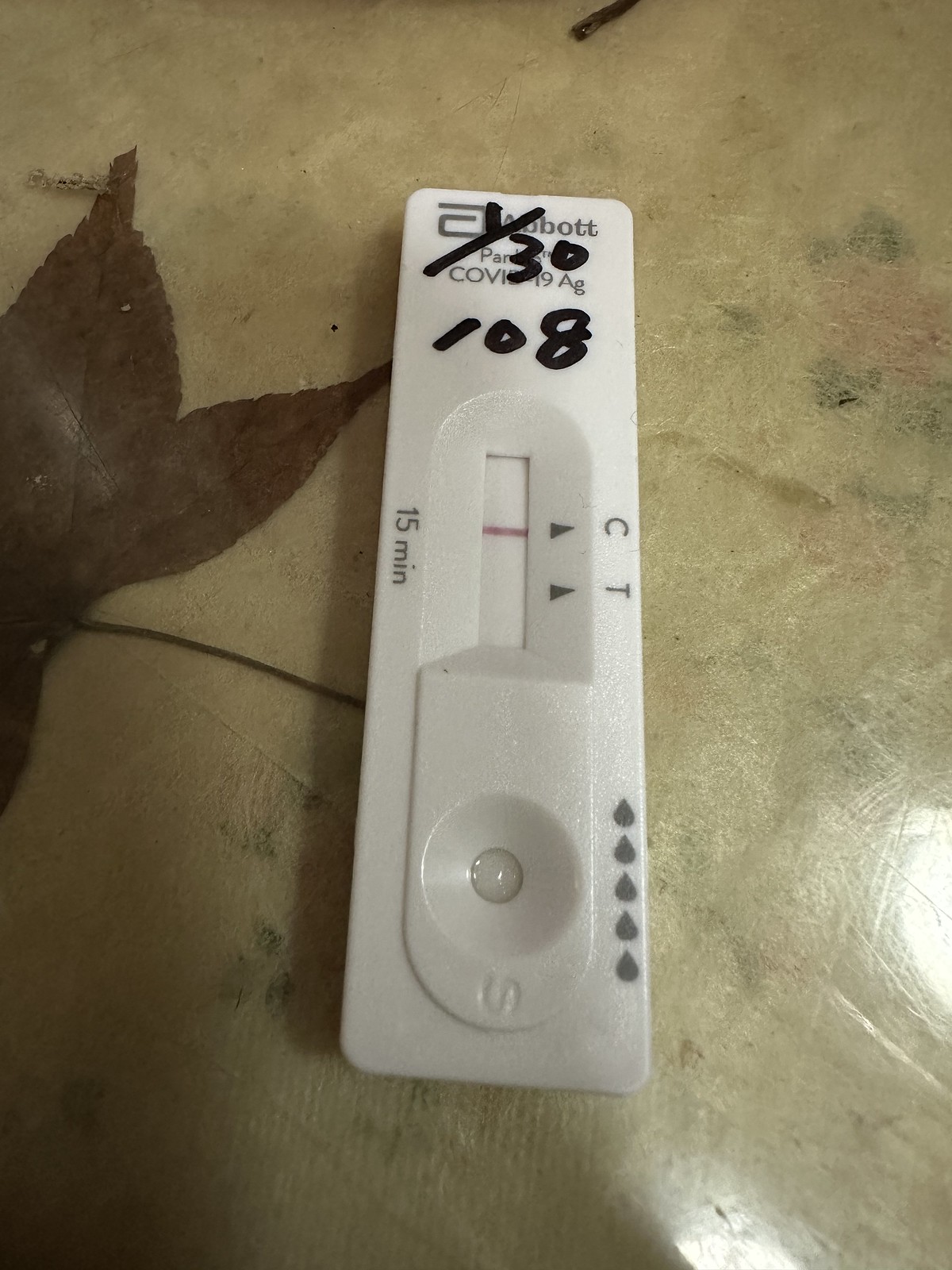An image depicting a COVID-19 test rests atop a glossy, gray-toned concrete floor. The floor's sheen adds an intriguing backdrop to the scene. In the left-hand corner, a black object resembling a mermaid tail or spread-out fish fin unfurls against the floor. Centered to the right, a white rectangular COVID-19 test kit draws immediate attention. The brand "Abbott" is inscribed at the top in black, accompanied by the word "COVID." A section appears to be marked with a black marker, displaying the numbers "130" followed by "108."

Central to the test kit, a rectangular window features the letters "C" and "T" at the top, each with arrows directing towards corresponding points. A prominent red line is visible beneath the "C," indicative of the test's result. As the eye moves downward, a circular indentation with a hole marks the bottom section, positioned above three small black dots. The bottom right-hand corner of the image captures two distinct light reflections, adding a layer of visual depth to the composition.